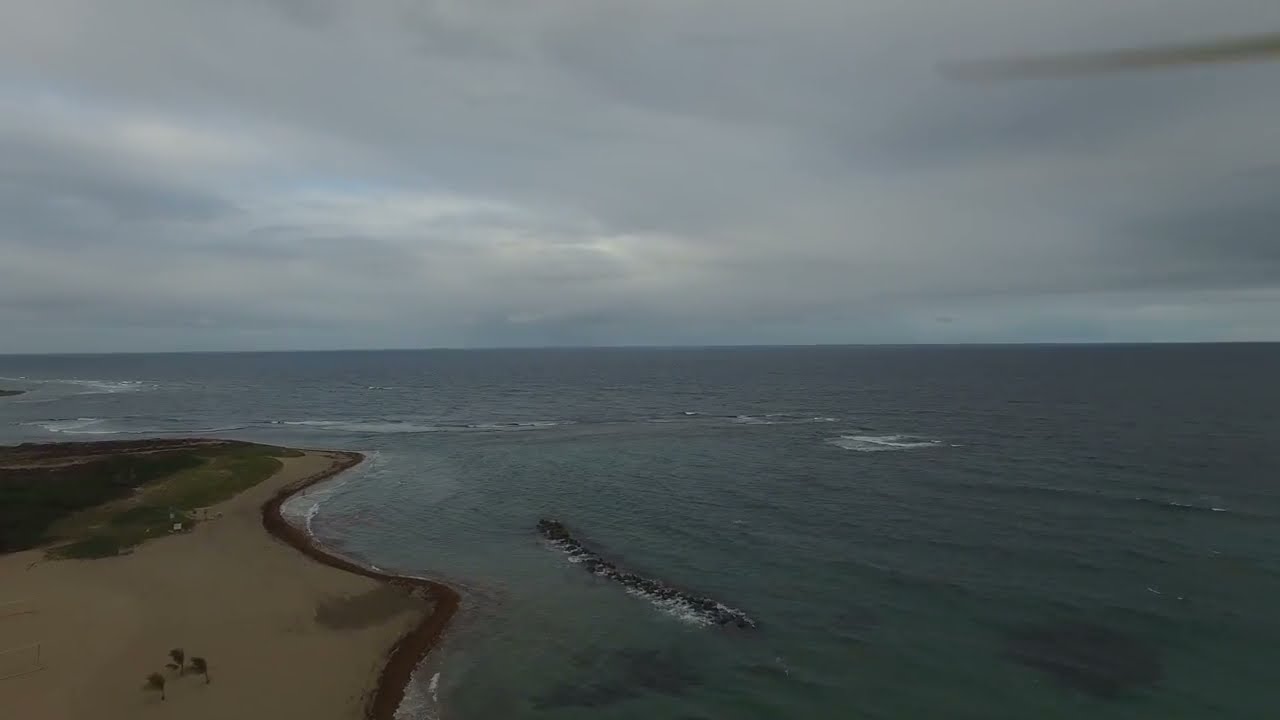This aerial image showcases a vast expanse of the ocean, characterized by its dark grayish-green waters punctuated with white-capped waves. The sky above is densely overcast with a mix of white and gray clouds, suggesting an early morning or late afternoon setting, possibly prelude to a storm. On the left side of the image, a stretch of tan and brown sand beach is visible, bordered by patches of green grass and three small palm trees. The coastline near this beach extends slightly into the water, forming a minor peninsula or island-like area. The horizon line is clearly defined, where the cloudy sky meets the endless sea. The scene is predominantly somber and serene, with minimal sunlight breaking through the thick clouds.